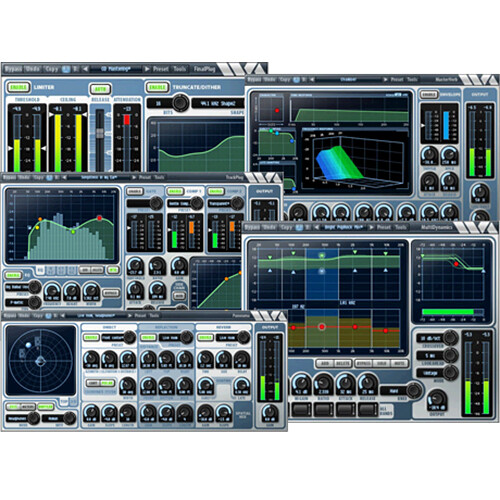The image is a screenshot displaying five technical instrument interfaces, reminiscent of music production plugins, layered and overlapping within a single frame. The primary color scheme consists of silver, blue, green, and yellow. In the upper left corner, the first screen features vertical green-to-yellow bars indicating measured data. Adjacent to the right, the second screen displays various wavelength diagrams, with undulating lines running horizontally. Below it, another screen presents similar wavelength diagrams, with lines extending left to right and fluctuating vertically. The bottom left screen appears to be a radar or sonar map, depicted as a circular bullseye with a dot indicating a specific location within the target area. The top-most screen on the left integrates a series of knobs alongside multiple charts and graphs, including square and 3D types. Overall, the screens are filled with detailed data indicators, charts, and knobs, suggesting a highly technical context that could apply to various professional fields beyond sound measurement.